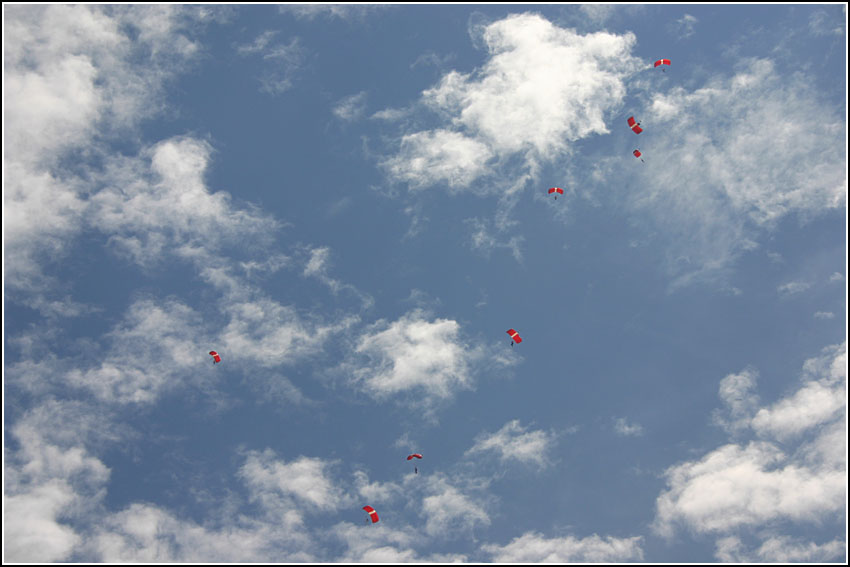In this vivid, color photograph, eight skydivers are captured mid-descent, their parachutes opened against a vibrant blue sky dotted with wispy white clouds. The skydivers are strategically arranged, mostly forming a diagonal line from the bottom left to the top right of the image, with one skydiver centered horizontally to the far left. Each parachute is distinctive, featuring a red canopy with a prominent white stripe running horizontally across the middle. The contrast between the rich blue sky and the red-and-white parachutes creates a visually striking composition. The sky is clear without any indication of impending bad weather, making the day perfect for skydiving. Sparse, wispy clouds break towards the center of the image and are denser in the left and bottom right sections, with a notable large cloud in the top right. The scene, likely from a skydiving exhibition or a group skydive, emphasizes the serene and exhilarating nature of the sport on a beautiful, clear day.